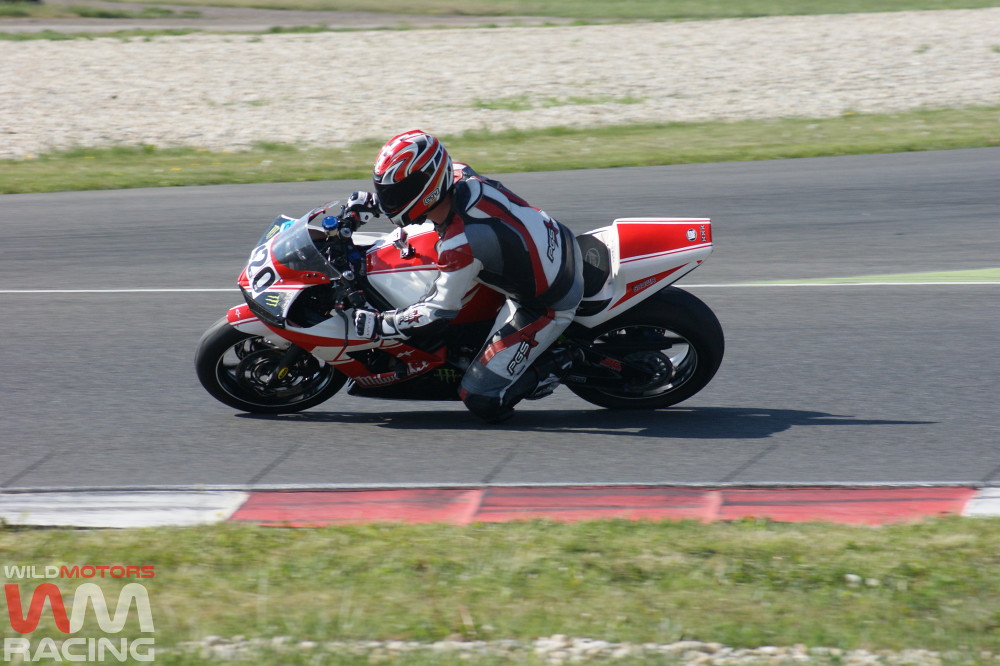This image captures the thrilling moment of a motorcycle racer, rider number 20, navigating a sharp left-hand turn on a racetrack, his knee skimming just above the pavement. The rider is dressed in a coordinated outfit with red and white stripes, matching his red and white motorcycle. His helmet, predominantly red, white, and gray with a black visor, complements the sleek design of his racing gear. The racetrack itself is bordered with red and white markings and features a grassy area nearby, indicative of a professional racing environment. This photo, taken at a Wild Motors WM Racing event - identifiable by the logo in the bottom left corner - highlights the speed and precision of the racer, who appears to be isolated on the track, emphasizing his focus and the intense nature of the sport.